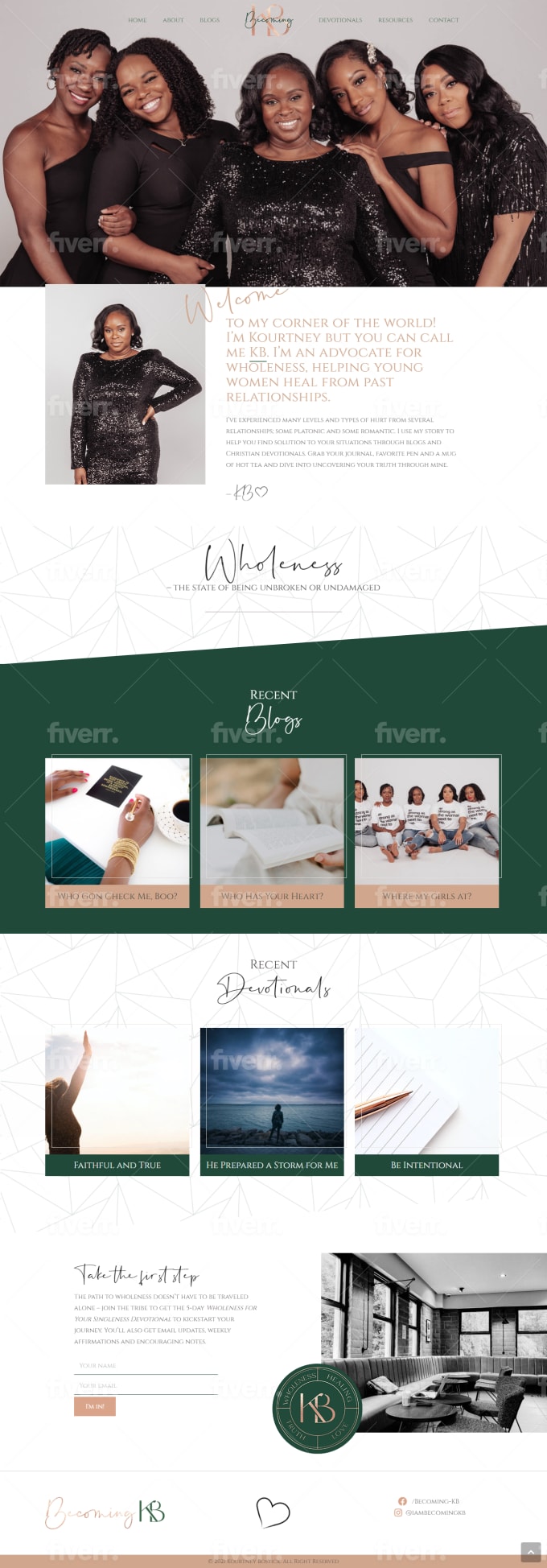The image depicts a webpage with a vertical layout, approximately three times as high as it is wide. At the top, occupying around 20% of the total height, is a banner showcasing five Black women in their 20s and 30s. They are all smiling and dressed in various black dresses, forming a close group as they lean towards each other. The women are visible from the hips up. Above them, there is faint, somewhat unreadable text that seems to outline the website's menu. Centered above the group is a logo in black cursive writing, though the text is not legible.

Below this banner, on the left side, there is an image of another Black woman in a black dress, directly facing the camera. To the right of her image is a block of text in golden font, which transitions into smaller black text, accompanied by a signature below, suggesting it might be a personal message or a quote.

Further down the page, another banner, roughly 20% of the page's height, features a dark hunter green background. This section contains three different images. The rightmost image features a group of Black women dressed in white t-shirts and jeans, seemingly younger in age.

The overall aesthetic of the webpage combines formal and casual elements, focusing on a cohesive theme centered around Black women.